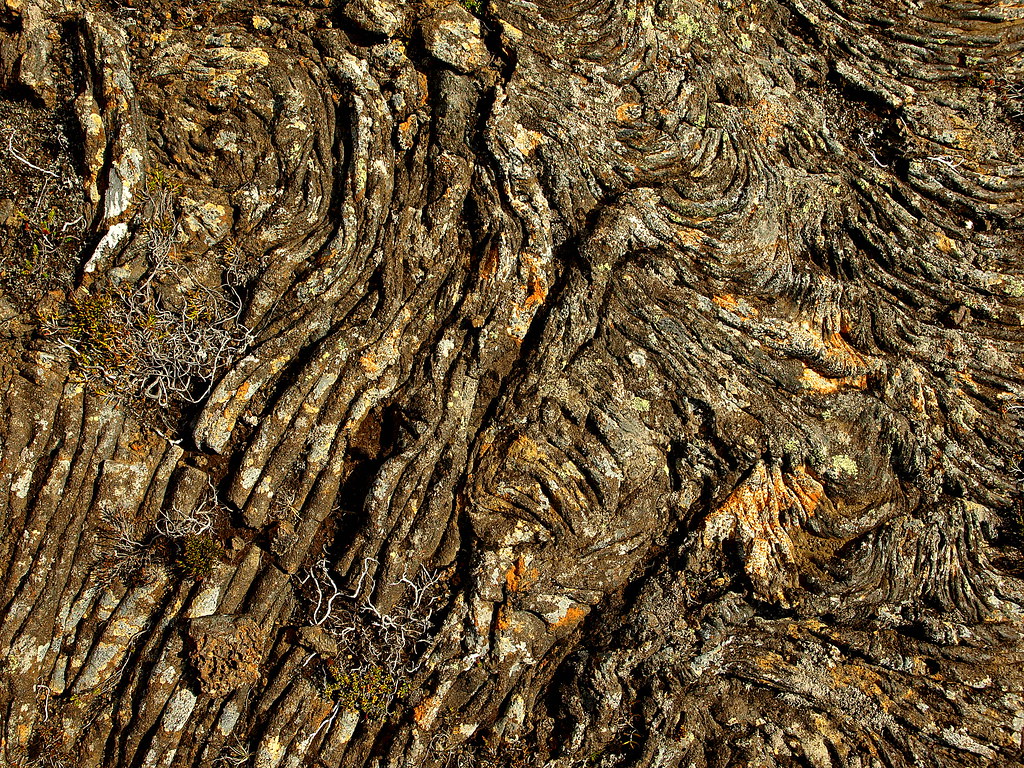A close-up image of tree bark with a deeply textured surface featuring intricate wrinkles that swirl, twirl, and ripple in all directions. The bark, a rich brown color, showcases a natural marbling of gold and orange hues. Various growths including moss, lichens, and small patches of soil cling to its surface, adding layers of texture and color. Some sections of the tree bark reveal the bare trunk beneath, where the wrinkles have been worn away. There's an appearance of aged wisdom and natural artistry, making it a truly fascinating specimen of an old, weathered tree.